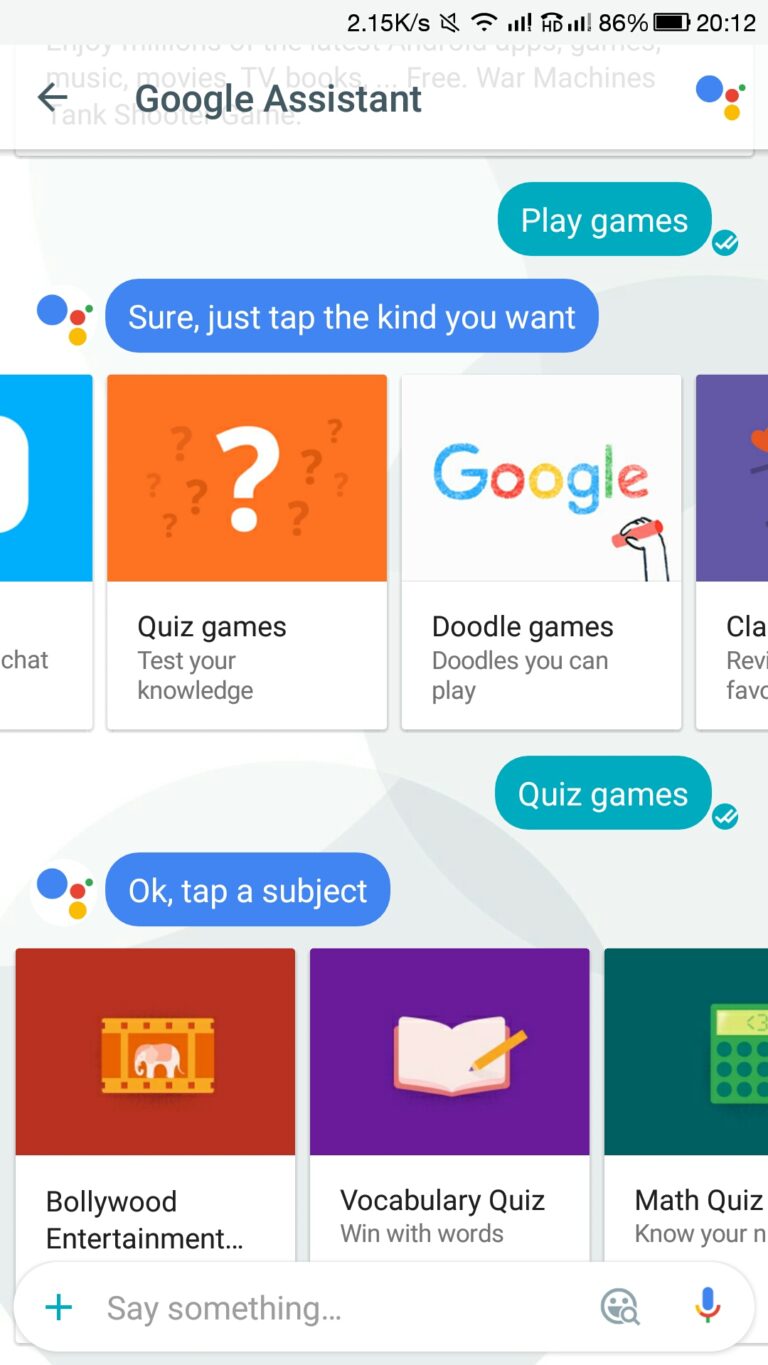This image is a screenshot taken from Google Assistant on a smartphone. The top section displays various status icons, including the time at 20:12 (8:12 PM) on the right side, along with a battery level indicator showing an 86% charge and Wi-Fi connectivity symbols. Notably, there are no icons on the left side of the status bar.

In the main content area, a user interaction is depicted. The user has typed “play games” into the input box on the right, presented in a teal speech bubble. Google Assistant responds in a blue speech bubble, stating, "Sure, just tap the kind you want."

Below this conversational exchange, there is a scrollable menu showcasing different game categories. Each category is represented by a colored square icon with related imagery. One prominently visible category is "quiz games," symbolized by an orange square containing multiple question marks, one of which is white. Other visible categories include "Google Doodle Games."

Further down, the user refines their request by typing "quiz games" again, prompting Google Assistant to suggest specific quiz topics: Bollywood, entertainment, vocabulary, and math quizzes. The interaction area concludes with an input prompt, "Say something...", allowing the user to continue their conversation with the Assistant.